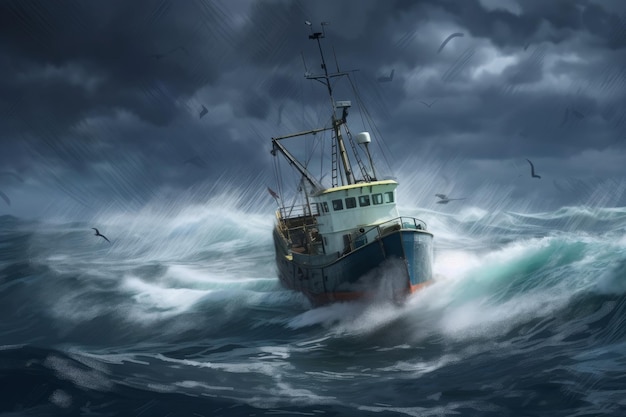This striking painting vividly captures a turbulent sea under dark, stormy skies. The central focus is a small trawler or tugboat, distinguished by its blue upper hull and red anti-fouling paint on the bottom. Positioned slightly off-center and pointing toward the lower right, the boat is navigating through aggressively high waves topped with whitecaps. The detailed depiction includes the masthead, radar, radio antennas, ropes, winches, and a surrounding railing. The sky is densely packed with dark, rolling clouds, while the ocean itself is a blend of dark greens and blues, churning with white foam and spray. Several seagulls or dark birds, about six in number, are visible flying on either side of the boat. The painting, likely oil-based, achieves a photorealistic effect, emphasizing the dramatic, almost gloomy atmosphere of a fierce storm at sea.